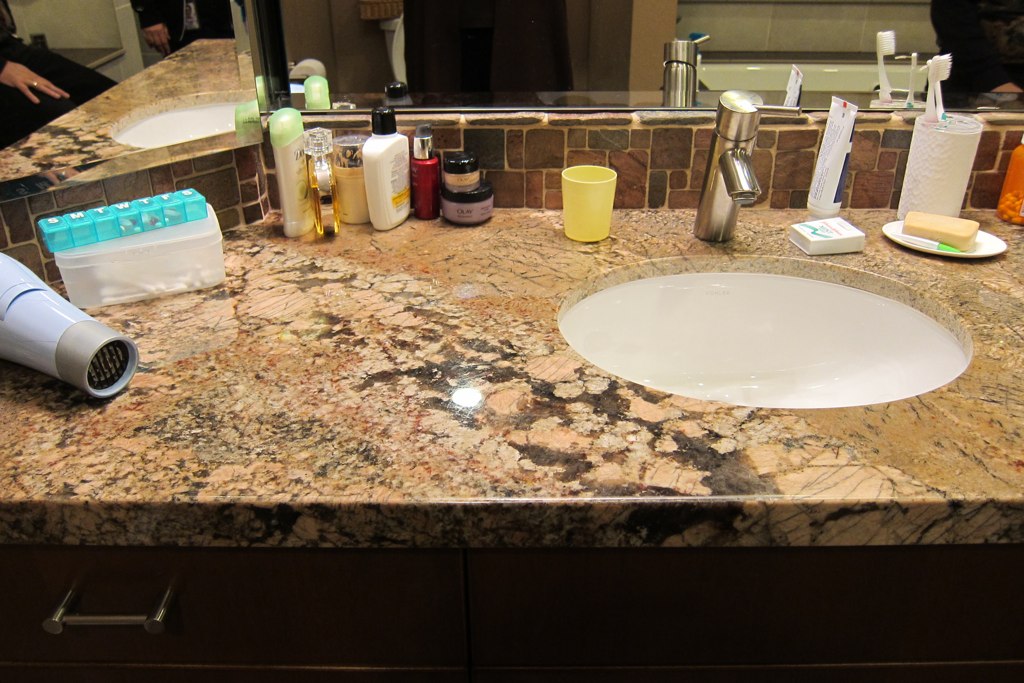This image captures a close-up view of a meticulously arranged bathroom sink and its surrounding countertop. The sink itself is almost round, slightly leaning towards an oval shape, and its bowl gleams a pristine white. Looking from the left side, the stone countertop showcases a polished surface of natural tan and dark brown tones, adding a touch of elegance to the setting. At the center lower left, a small white spot of reflection can be seen on the countertop. 

To the left of the sink, a gray hair dryer with a dark gray nozzle rests. A pill container marked with the days of the week (SMTWTFS) shows pills stored in the Wednesday, Thursday, and Friday compartments. Below the pill container lies a transparent plastic vessel. Next to it, an off-white deodorant with a light green cap stands. Several other personal care products occupy the space, including a rectangular bottle with a black cap, and a nail polish bottle characterized by a silver cap and a vibrant red body. Two cylindrical makeup containers, one stacked atop the other, feature a black cap and tan base for the top container, and a black base with a lavender body for the lower. 

Adjacent to the polished sink spout, a smaller yellow cup sits, while immediately to the right of the faucet, a dental floss container lies on its side next to a tube of toothpaste whose logo is not visible. A toothbrush holder, designed as a cylinder, contains two toothbrushes. A nearby soap dish holds a bar of tan soap, accompanied by a white and green cylindrical item positioned in front.

The background reveals dual mirrors: one positioned on the right and the other on the left. In the mirror on the left, the sink is again visible, along with the reflection of a woman's hand adorned with a ring on her ring finger. This intricate scene paints a detailed and vivid picture of a well-used and organized bathroom space.